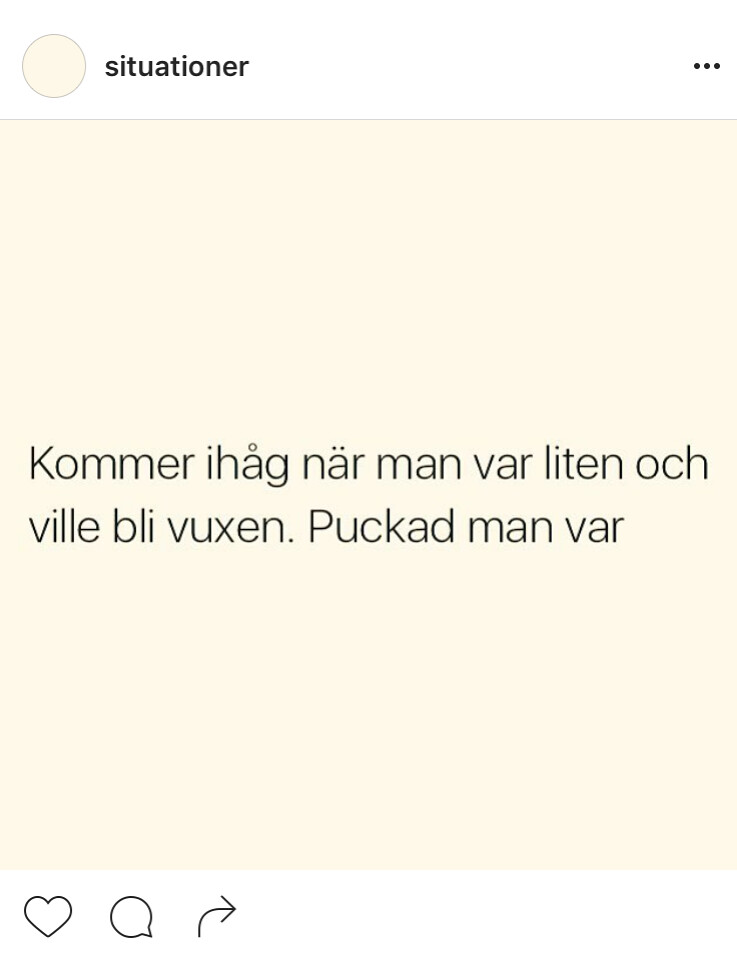The image appears to be a simplistic Instagram post displayed on a cell phone, sporting a minimalistic design. At the top left corner, there is a cream-colored circular profile icon next to the username "situational" in lowercase letters, though another description spells it as "Situationer" in uppercase. Directly across on the top right, three horizontal dots form a hamburger menu for additional options.

The main content is centered within a square, pale pink background, featuring black text in a non-English language, possibly Dutch or a Scandinavian language. The text reads: "Komir ihag naar maan vaar liten och vil bli vuxen pokad maan vaar."

Below the main image, common social media interaction icons are lined up left to right: a heart for liking the post, a speech bubble for comments, and a curved arrow for sharing or sending the post.

All elements come together to create a basic, yet easily recognizable Instagram post layout.